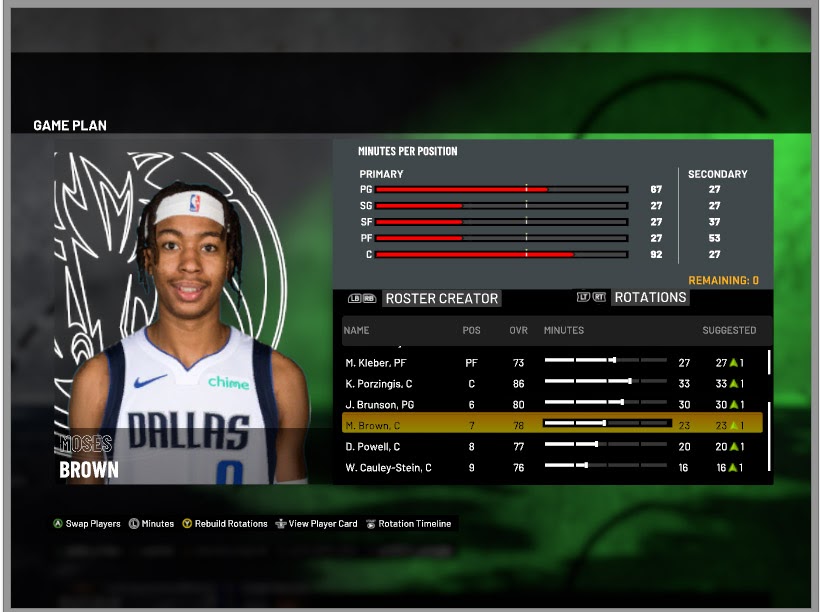In this detailed and descriptive caption for the image:

A striking sports-themed image, potentially sourced from a platform like ESPN, showcases a young basketball player prominently featured in the center. The background is a dynamic blend of black, gray, and green hues. Above the young man's face, the bold, capitalized text "GAME PLAN" immediately catches the eye. The player is in front of an emblem, giving the composition a structured feel.

The player is wearing a white Dallas Mavericks jersey, complete with the iconic red and blue NBA logo, a Nike logo, and a Time Bank sponsor logo, which might indicate that he plays at the NBA level rather than college. The young man, likely between 18 to 22 years old, sports a white headband and has braided hair, along with a warm, youthful smile on his face. His appearance includes an African-American complexion, a mustache, and braids.

His jersey displays the name "Brown" on the back. The lower part of the image features various graphics and menus, such as "Minutes," "Restoration," and "View Player Card," indicating his in-game statistics and roles. Additionally, there are graphical bars depicting his stats, and beneath those, options such as "Roster Creator" and "Rotations."

Highlighted in the roster list is "Brown," among other names including Khyber, Perringis, Brunson, Powell, and Cully Scott, indicating the player is key in the lineup. This visually rich and information-packed image encapsulates the player's role and contributions to the team.